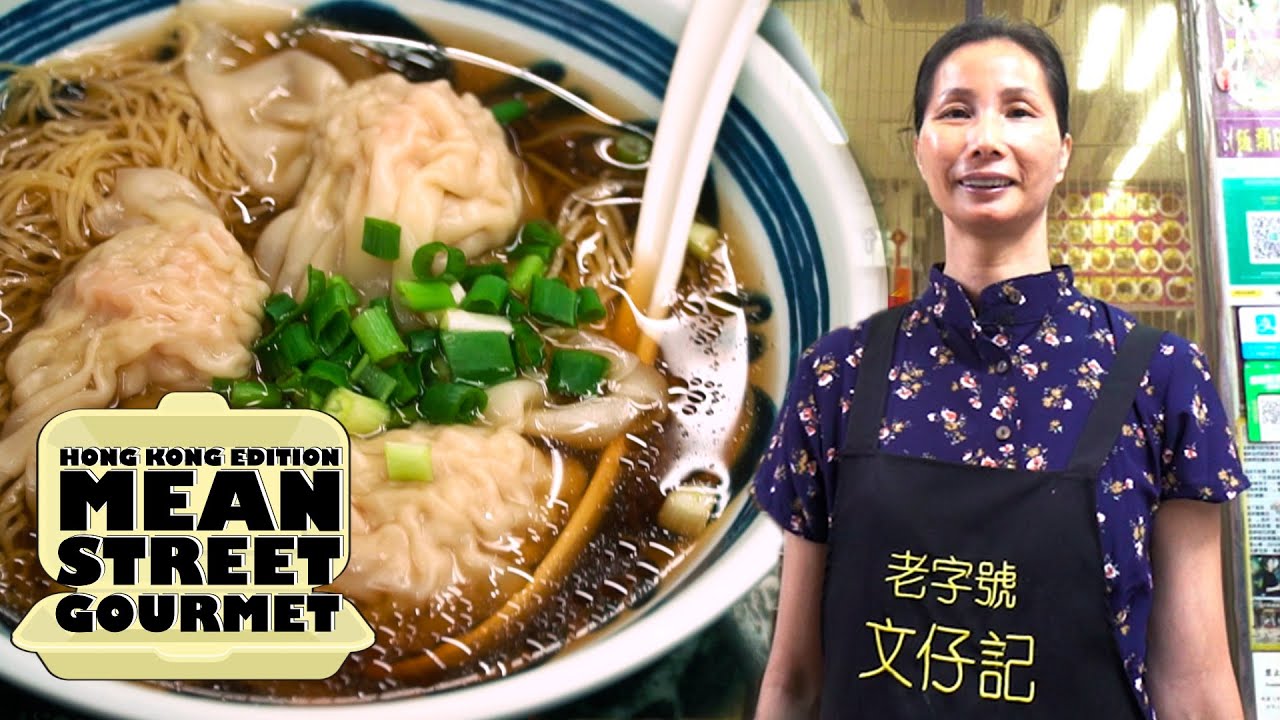The image is a detailed collage featuring a tantalizing bowl of noodle wonton soup as its focal point. The clear, light brown broth, slightly translucent with a hint of oil, cradles thin, yellow egg noodles and three large wontons with visible pink filling. Garnished with chopped green onions in the center, the soup is served in a white ceramic bowl with a blue patterned border. A plastic spoon is poised dipping into the rich broth. To the right of the bowl stands a middle-aged Asian woman, likely the chef, smiling with her hair pulled back. She is wearing a blue, high-collared shirt adorned with pink floral patterns and a black apron featuring yellow Chinese characters. The background subtly hints at a restaurant setting with some menu graphics visible. At the bottom left corner of the image, an open takeout box graphic prominently displays the words "Hong Kong Edition Mean Street Gourmet."